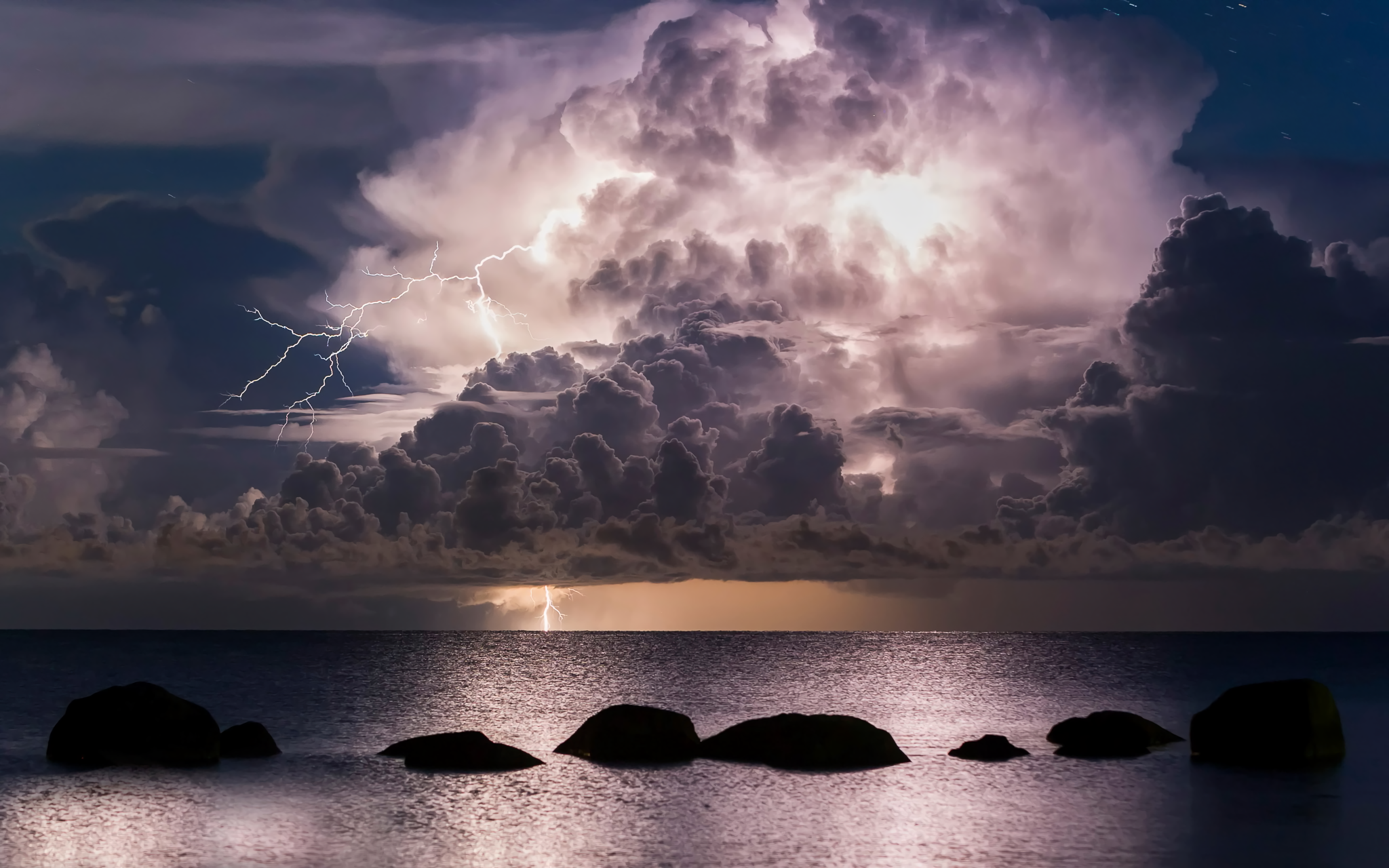In this striking color photograph taken at night, the intense drama of a coastal storm is captured. The scene overlooks the dark blue, nearly still ocean, where five low-lying rocks are silhouetted in the water, forming a horizontal row in the foreground. The water mirrors the dazzling display of the sky above, reflecting the bright, jagged lightning bolts that split the heavens and strike down toward the sea.

Dominating the upper two-thirds of the image is a tumultuous sky, composed of massive, dark gray clouds interspersed with lighter, puffy white clouds. These clouds swell upward and outward, creating a layered and textured backdrop. Amidst this chaotic skyscape, lightning bolts fork and dance, illuminating the scene with sharp, white and orange flashes. A particularly intense bolt can be seen extending prominently from one of the denser cloud formations. 

To the right side of the image, some trees are faintly visible in the mid-ground, adding another layer of depth to the scene. The overall composition creates a powerful contrast between the foreboding, stormy sky and the calm, reflective surface of the ocean below.